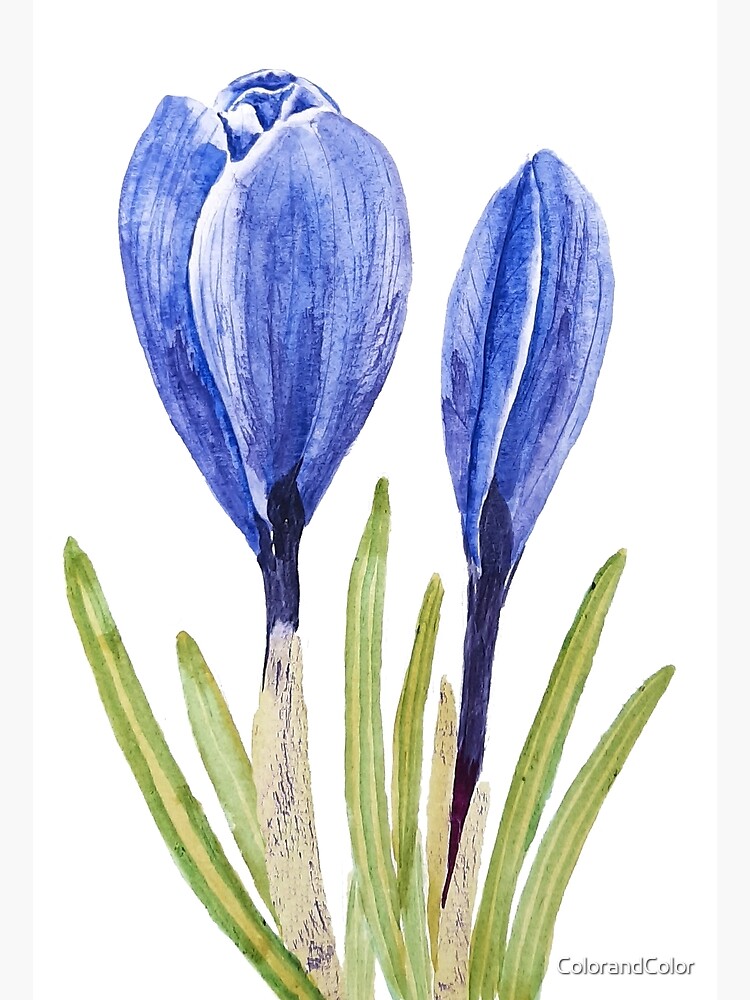This detailed watercolor painting, created on white paper, showcases a plant with two emerging, bluish-purple flowers. The flowers, situated on separate stems, exhibit a gradient with their bases transitioning from white to dark blue. Each flower has intricate edges of white, adding to their delicate appearance. The flower on the left is slightly more open than the one on the right, which remains tightly closed. The stems rise from a base of light green leaves, some of which feature a central yellow-to-tannish brown stripe, adding depth and variation to the foliage. Long, slender, brownish-green leaves intermingle with the stems, suggesting a natural withering effect. At the bottom left corner of the image, the word "color" is repeated, hinting at the artist's emphasis on the vivid hues throughout the artwork.